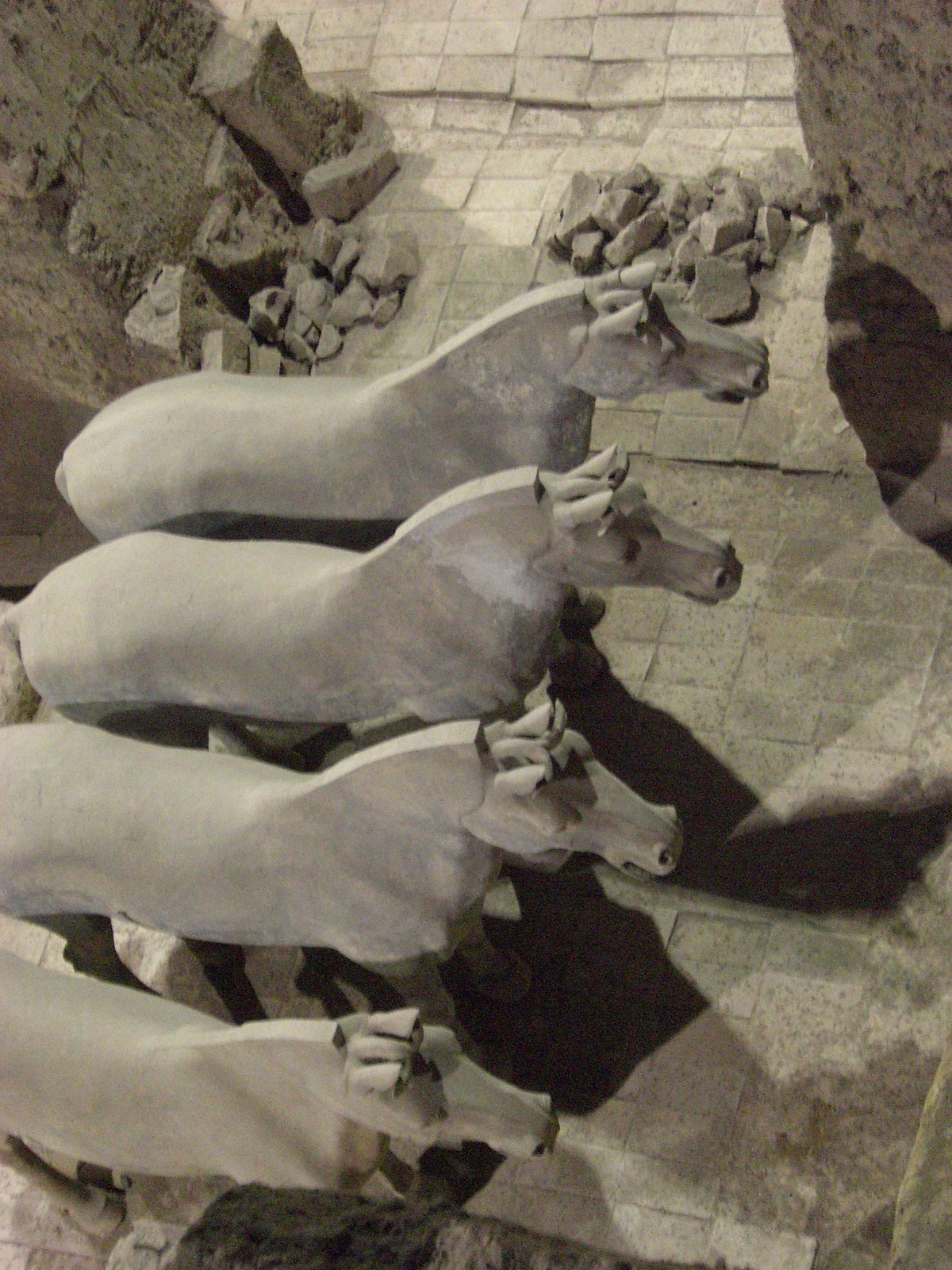This image, captured from a slightly elevated vantage point perhaps just a second story, offers a compelling aerial view of a courtyard dominated by four stone horse sculptures. These horses, each carved from light tan stone with subtle brown hues, possess a smooth but unpolished texture, giving them an ancient, enigmatic aura. The horses are uniformly aligned on the left side of the image, with their well-defined, basic outlines revealing short cropped manes, pointed ears, and slight locks of hair between their ears. Their serene yet alert poses, with forward-facing gazes and squared-off features, lend an unusual, almost ominous ambiance to the scene.

The horses are positioned against a backdrop of a courtyard floor paved with tan bricks, interspersed with areas of sand or clay that evoke an archaeological site. The photo cuts off parts of the first two horses, emphasizing their linear arrangement and contributing to the image’s depth. Above the courtyard, a door flanked by pillars hints at further exploration beyond the immediate scene, while areas of broken and crumbling bricks at the top convey a sense of faded grandeur.

In this detailed portrayal, shadows cast by the horses add a subtle variation in lighting, enhancing the texture and dimensionality of the image. The entire scene encapsulates a moment frozen in time, blending elements of artistry and history.